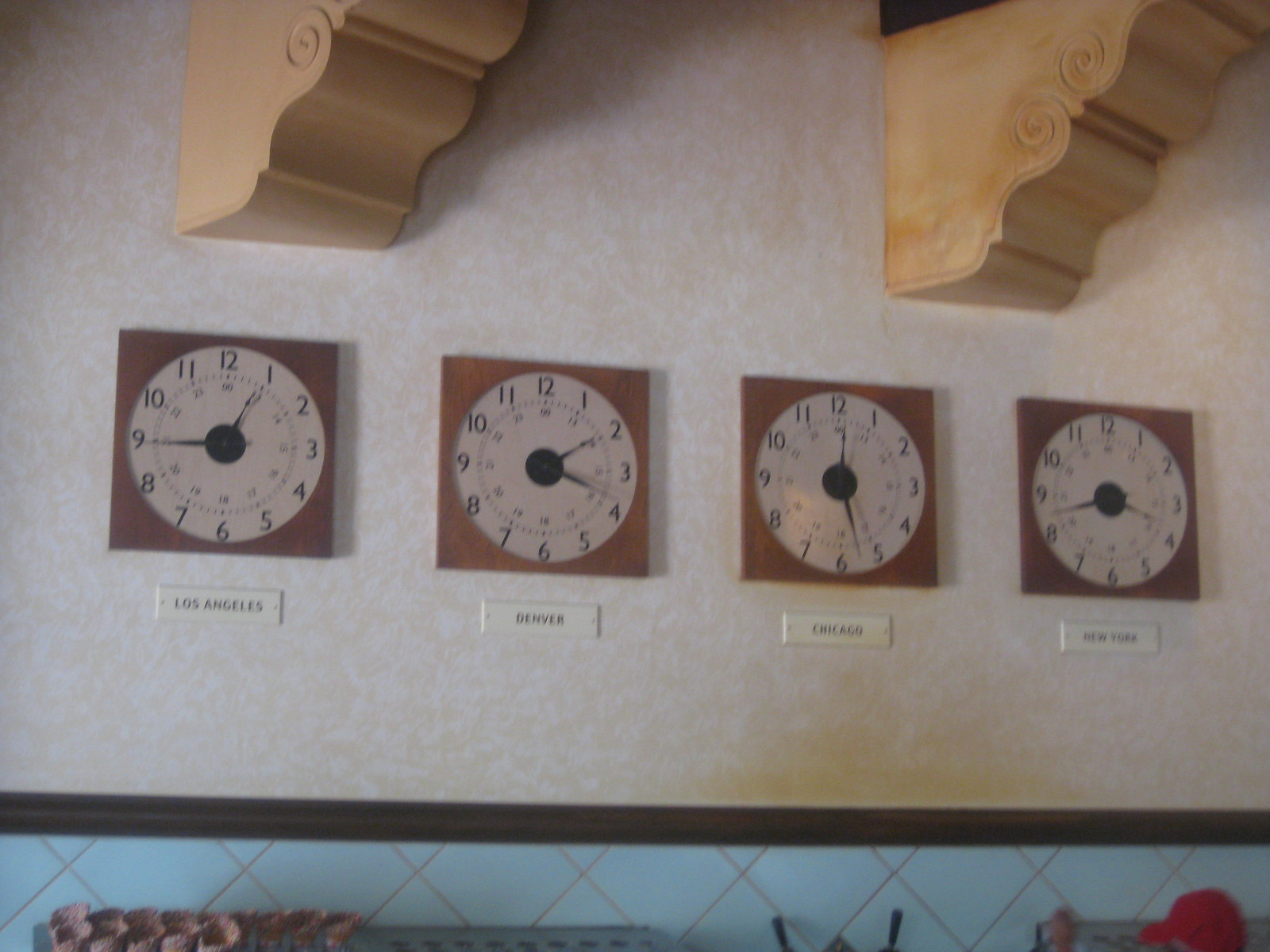The photograph captures a decorative wall adorned with four prominently displayed clocks, each marked with the city names Los Angeles, Denver, Chicago, and New York. The clocks feature round white faces with black numerals set within square brown wooden frames. Notably, the hour and minute hands across these clocks appear inconsistent and do not reflect accurate times. Above the clocks, two ornate, wedge-shaped wooden supports are present, hinting at the bottom edges of beams, adding a touch of elegance to the scene.

The wall itself is decorated in a pale white patterned wallpaper, complemented by a section of blue crisscross wallpaper with wooden trim near the bottom. There is a strip of what appears to be black beam running horizontally, above which the clocks are mounted. Lower down, the image shows a surface cluttered with various indistinct items, including something red that could be a hat or antenna, and a few shell-like objects in the bottom left corner. The overall ambiance of the room suggests a blend of classic and eclectic design elements.